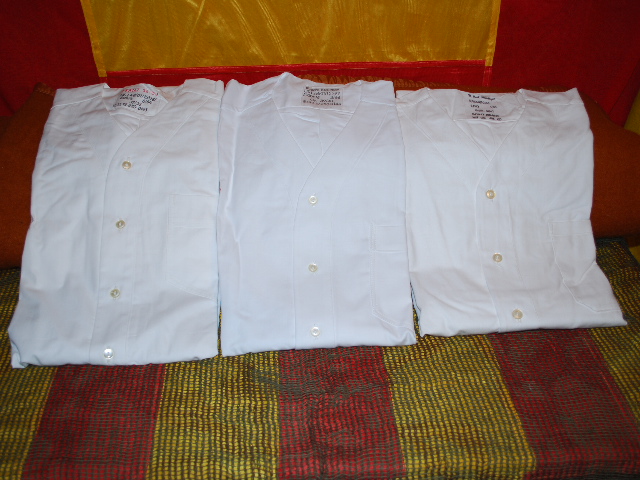This is a photograph of three neatly folded, white button-up shirts displayed in a row. Each shirt features yellowish clear buttons down the middle and a V-neck style at the top. They have tags with text in Japanese or Korean characters, indicating they might be part of a uniform. The shirts rest on a striped fabric bench or seat with red and yellow colors reminiscent of McDonald's, and they lean against a red pillow. Behind this setup is a decorative wooden headboard or wall. The image, captured in medium light with a slightly off focus, appears suited for listing these clean, new shirts for sale online.